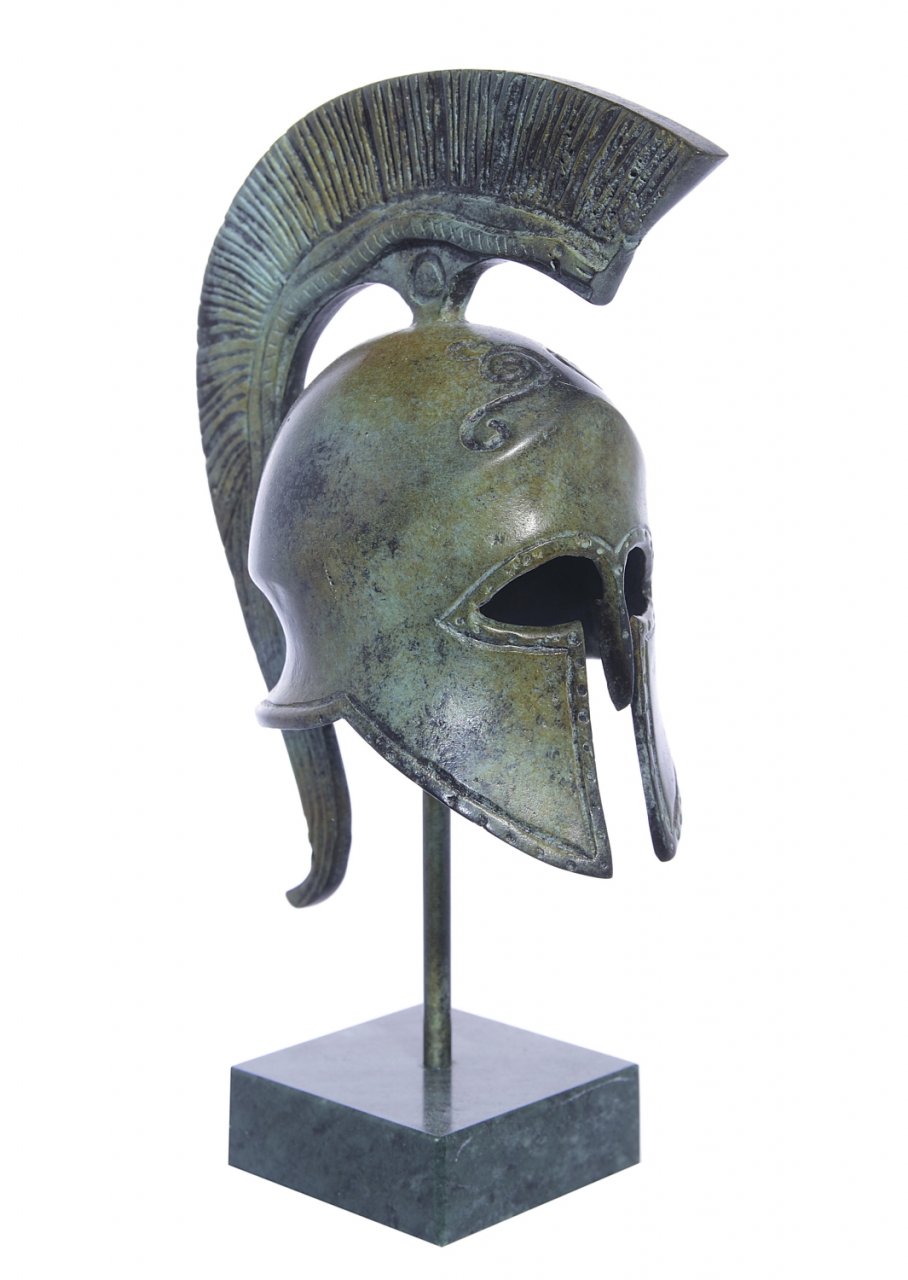The image depicts a detailed reproduction of an ancient Roman helmet, meticulously placed on a display stand. The helmet, crafted from metal with a dark jade hue accented by brown touches, covers the entirety of the head, from the back to the top, and features a prominent nose guard that descends between the oval-shaped eye holes. It also has large, triangular cheek protectors. Atop the helmet sits an impressive mohawk-like crest, resembling a brush or broom, which starts at the top of the helmet and extends down the back, curving gently at the neck. This intricate piece is mounted on a metal rod, which extends from a shiny, black marble base that reflects some of the helmet’s details. The helmet is oriented towards the right, slightly angled towards the viewer, enhancing its majestic and historic presence.